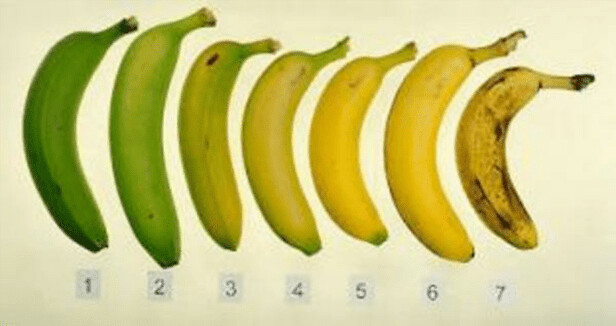This detailed illustration showcases seven bananas at various stages of ripeness, arranged from left to right and labeled numerically from one to seven. The background is a beige-white canvas, darker at the bottom left corner, giving the image a subtle contrast. The bananas transition from unripe to overripe as you move across the image. The first banana, labeled "1", is a dark, vivid green, resembling the color of a lime. The second, "2", is slightly larger and a medium green with hints of yellow. Banana "3" is primarily yellow with traces of green and a small bruise. Number "4" has green just at its tips, signifying it’s almost ripe. "5" is mostly yellow, with just a touch of green at the bottom, indicating it’s ready to eat. The sixth banana, brightly golden yellow with a few tan spots, is in prime eating condition. The seventh and final banana is yellow with multiple dark brown spots, clearly overripe and ready for banana bread. The image, although grainy and low in quality, serves an educational purpose by vividly depicting the stages of banana ripeness from unripe to overripe.